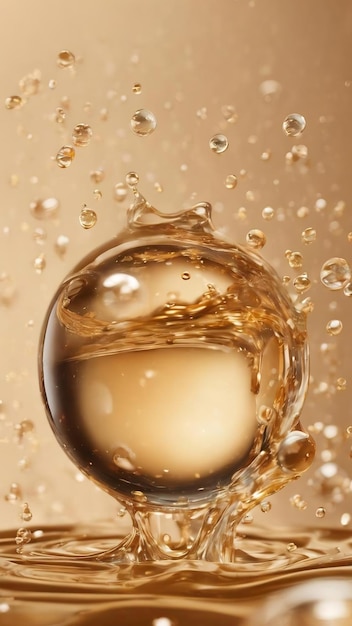The image illustrates a highly detailed and artistic close-up of a liquid splash, likely AI-generated, depicted in various shades of brown and champagne. Central to the composition is a glossy, bubble-like droplet that appears suspended in mid-air, with smaller glowing droplets scattered around it, reminiscent of tiny gemstones. The backdrop is a light brown gradient, complementing the darker brown hues of the liquid. The surface of the liquid below features small waves and ripples, suggesting disturbance, with some rising up towards the suspended central droplet. The entire scene, with its glassy surface and digital artistry, imparts a surreal and otherworldly quality, accentuated by the gradient and the intricate play of light and reflections.